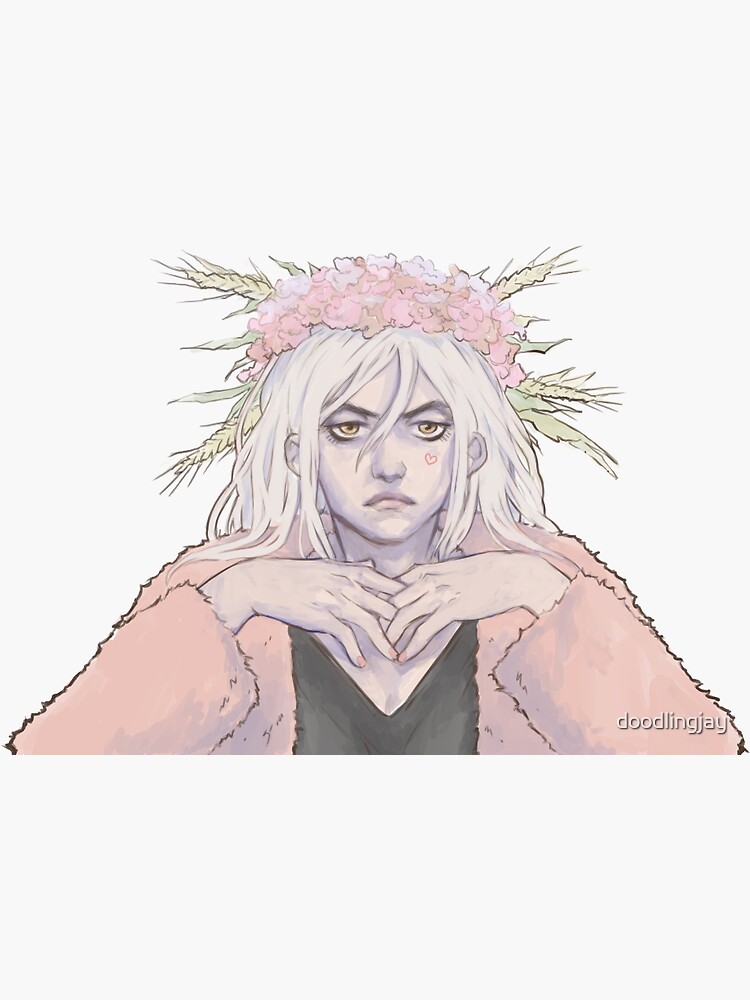This vertical illustration, titled "doodling J" as indicated in the bottom right corner, portrays a young girl with a melancholic and disgruntled expression. Rendered realistically with cartoonish elements, the girl's long, light blonde almost white, slightly wavy hair cascades around her face, with some bangs tucked behind her ears revealing her ears. Her sad brown eyes, adorned with dark eyeliner, gaze intensely with half-closed lids, highlighting her unhappiness. She has a small red heart tattoo just below her left eye and her mouth turns downward in a frown. 

She wears a fuzzy, pastel pink jacket over a black v-neck shirt, adding a touch of subdued color to the otherwise pale and light-toned palette of the image. Her hands rest just below her chin, with fingers interlaced, displaying painted nails. Adorning her head is a floral crown composed of pink and dark pink flowers, wheat fronds, and green leaves, enhancing the delicate and somber mood of the illustration. The background is stark white, centering full attention on the girl's downcast figure, which is seen from the shoulders up.